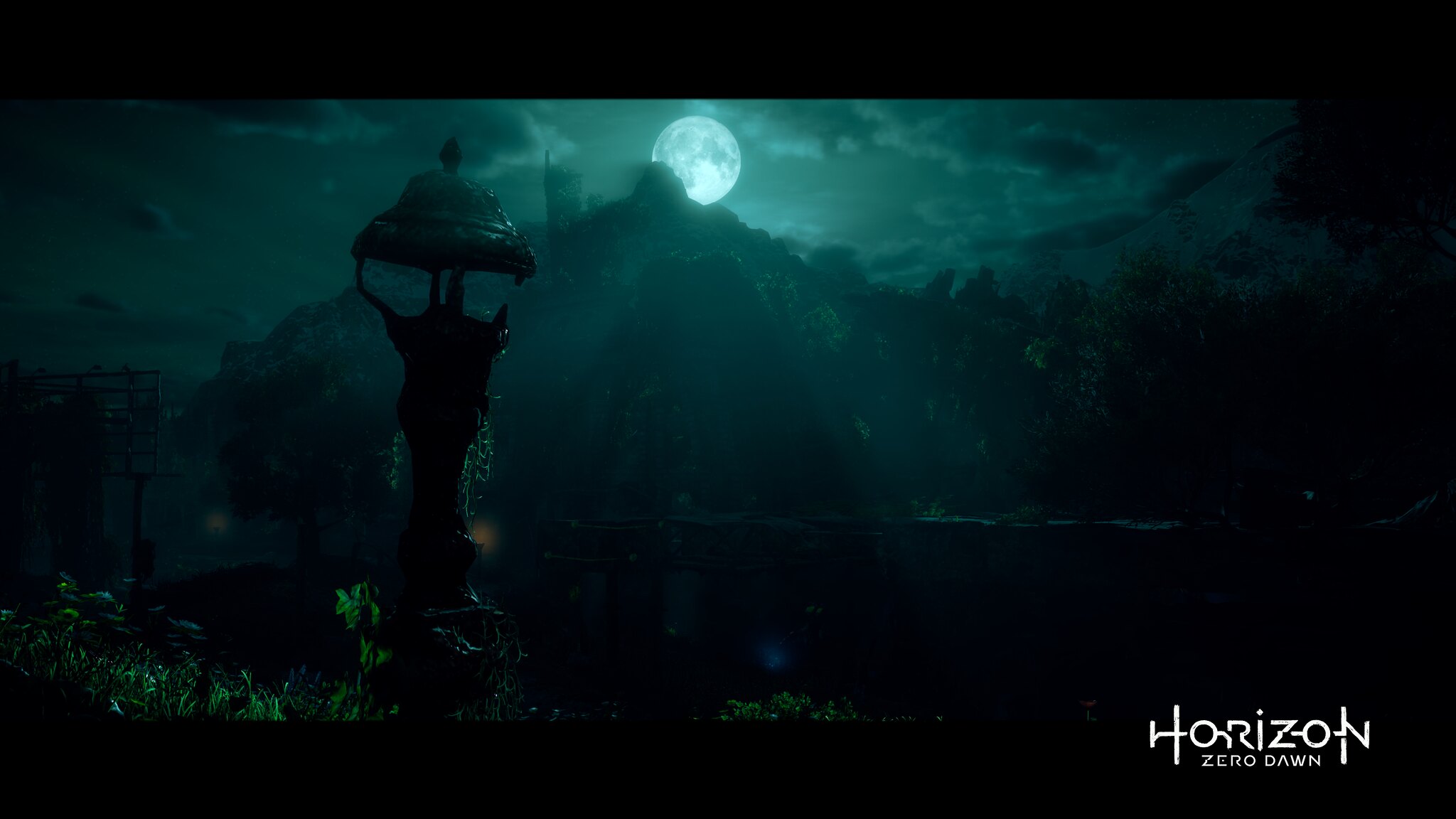The image portrays a hauntingly dark scene, evoking a sense of foreboding. A singular, ominous black hill dominates the background, silhouetted sharply against the glow of a full moon. Visible upon the moon's surface are faint images that resemble a castle or a tall, enigmatic structure, adding an otherworldly element to the scene. In the foreground stands a broken street lamp, reminiscent of a vintage house lantern. The lamp is missing its glass panels, its top is bent, and it leans precariously. Ivy weaves up its post, mingling with surrounding tall grass and various plants. A mysterious red light emanates from the right side, adding an eerie hue to the darkness. At the bottom right of the image, the text "Horizon Zero Dawn" suggests that this eerie tableau is part of a video game, further enriching the narrative with a layer of intrigue and impending adventure.